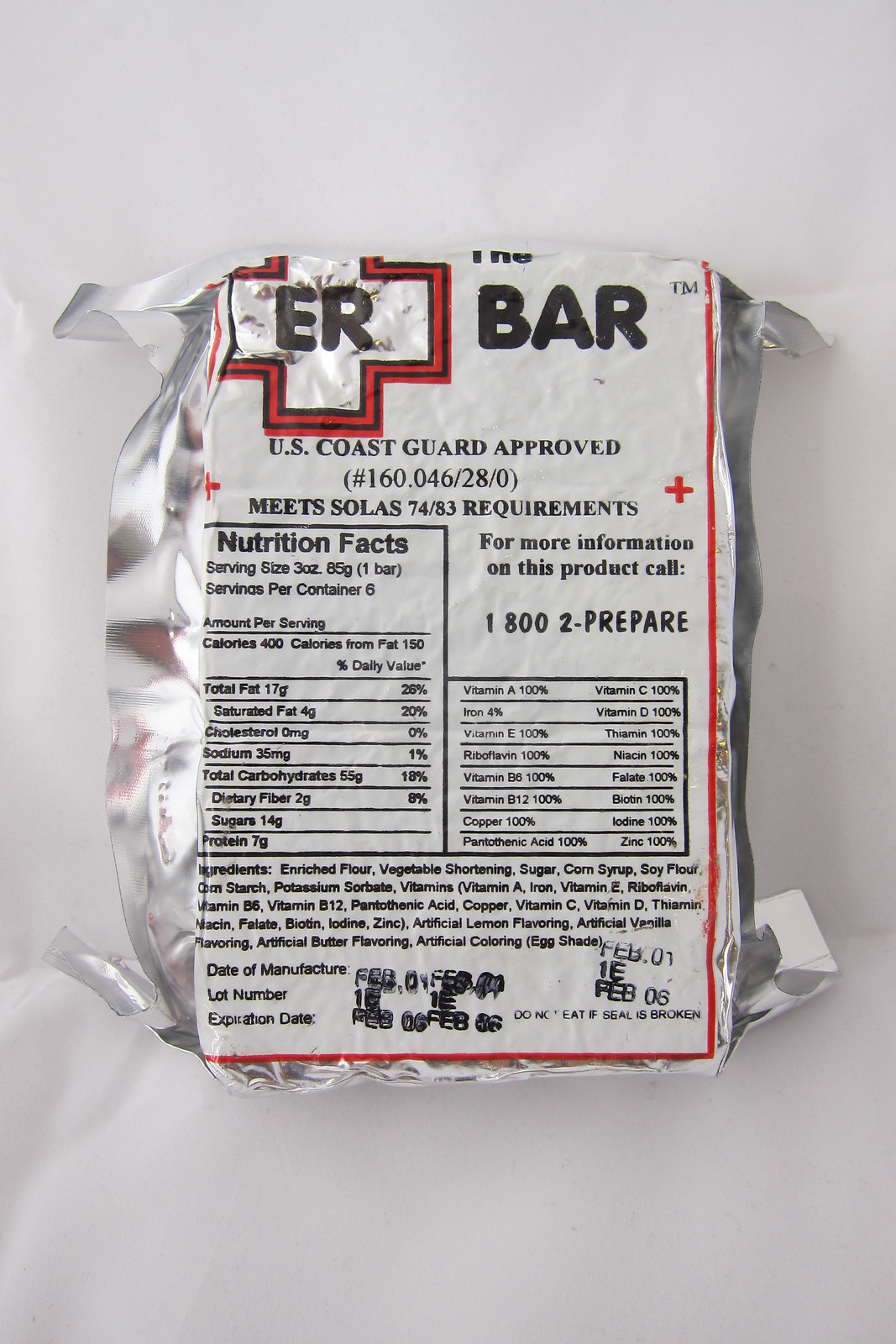The image showcases the back of an "ER Bar" wrapper. The label features a distinctive "ER" text styled within a red cross shape. Directly underneath, in black font, it states: "US Coast Guard Approved. Number 160.046-28-0." It also meets "SOLAS 74/83 requirements." 

On the left side of the wrapper, a boxed section presents the Nutrition Facts. The serving size is listed as three ounces (one bar), with a total of six servings per container. 

The right side of the wrapper includes additional information: for more details about the product, there's a customer service line, "1-800-2-PREPARE." Below this, the Nutrition Facts box continues, enumerating the vitamins and minerals contained in the ER Bar. 

Overall, the wrapper's design emphasizes its compliance with safety standards and provides comprehensive nutritional information and customer support details.